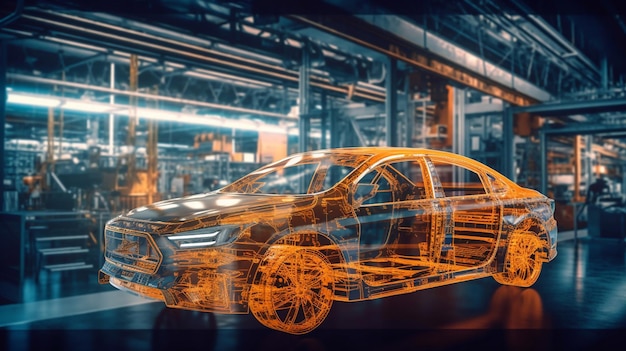The image depicts a high-tech, computer-generated illustration of a translucent sedan, rendered in bright orange. The car's webbed orange wheels and detailed orange outlines contrast sharply against its transparent body, through which a dark industrial setting can be observed. This setting includes a shiny black floor, a glass or mostly-dark factory interior accentuated with occasional orange pillars, reflective surfaces, and a black staircase. The scene emits a futuristic, high-tech vibe, reminiscent of advanced conceptual designs or blueprints set within a sleek, modern workspace.